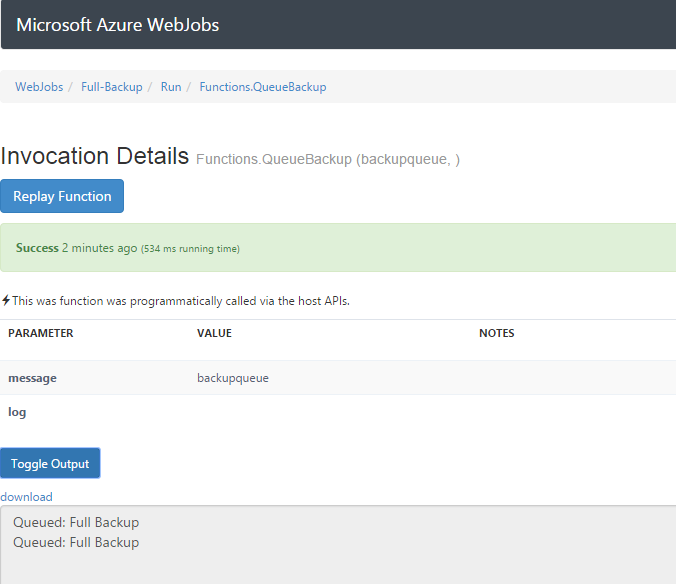In this screenshot, we see a page from the Microsoft Azure WebJobs interface dedicated to automating backups. The page title, "Microsoft Azure WebJobs," is prominently displayed in the top left corner. Below the title, four links are shown in blue font: “WebJobs,” “Full Backup,” “Run,” and “Functions to Backup.” 

Centrally located within the screenshot, there are detailed status updates, including metrics like "Success two minutes ago." Furthermore, below these updates, the interface indicates that these records are messages. 

The interface also features two blue buttons: "Replay Function" and "Toggle Output." At the very bottom of the page, there is a note that states, “The following was downloaded: queued full backup.” The entire page has a clean white background, emphasizing the functionality for automating backups on Microsoft Azure WebJobs.